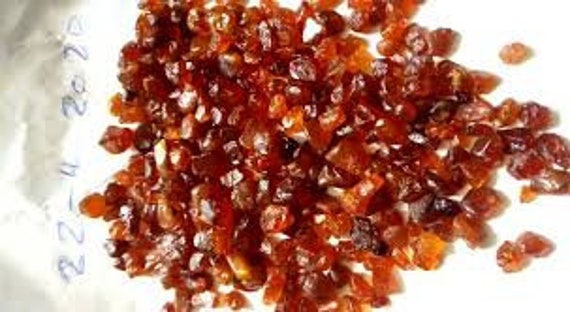The up-close image showcases an abundant collection of small, chewy-looking objects, primarily clustered in the center of the picture. The objects, numbering in the hundreds, range in color from dark reds and blacks to oranges and yellows. These pieces, possibly dried apricot, fruit snacks, or even amber, are displayed on a white background. A date, "22-4 2020," is written in blue on the left side of the image, adding context. Whether these objects are seeds, dried fruits, or fragments of amber remains indeterminate, but their vivid colors and varied sizes create a visually intriguing scene against the likely paper or plate background.